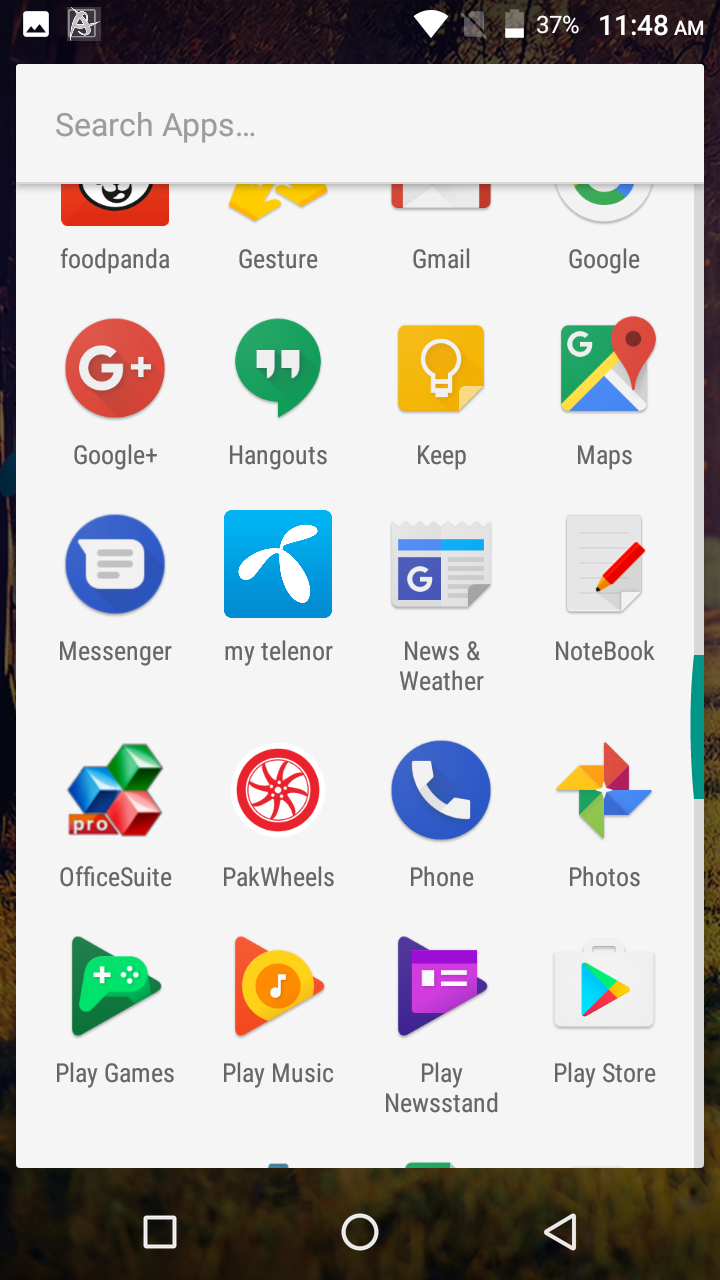The image depicts a smartphone screen in portrait mode featuring a variety of applications arranged into a grid-like pattern. At the top of the screen, there are typical smartphone status indicators: on the left, a small icon suggesting a Camera or Image Gallery is present, while on the right there are symbols for cellular reception, battery life at 37%, and the current time displayed as 11:48 a.m. Below these icons is a search bar outlined in white with the placeholder text "Search apps" in gray.

The main portion of the screen showcases an array of app icons. Notable among them are:

1. **Food Panda** - Presumably a food delivery service.
2. **Gesture App**
3. **Email** - For electronic mail.
4. **Google** - The primary Google app for search and other functions.

Additional specialized Google apps are also visible:
- **Google+** - Represented by a red circle containing a white 'G' and a plus sign.
- **Google Hangouts** - Featured as a green speech bubble with white quotation marks inside.
- **Google Keep** - Displayed with a yellow background and a white light bulb icon.
- **Google Maps** - Presumably for navigation.

Further down, there are more apps for various utilities and services:
- **Messenger**
- **My Telenor** (likely a telecom service provider)
- **News and Weather**
- **Notebook**
- **Office Suite**
- **PakWheels**
- **Phone**
- **Photos**
- **Play Games** - Represented by a green arrow intertwined with a game controller icon.
- **Play Music**
- **Play News Stand**
- **Play Store**

At the bottom of the screen, common navigational icons are visible: a circle (possibly the Home button), a square (likely for Recent Apps), and a left-pointing arrow (Back button). These are positioned on the right side, in alignment with typical Android user interface design standards.